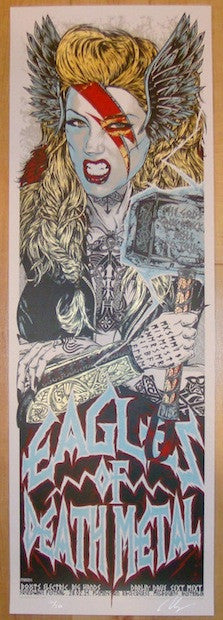The image appears to be a tall, thin concert poster with a white border and a thin gold frame around the edges, which is set against a light-colored background. Dominating the top part of the poster is the face of a fierce warrior woman, reminiscent of the Marvel character Thor. She has blonde hair, styled to fall both in front of and behind her shoulders, and striking, wing-like appendages sprouting from her ears. She glares forward with her teeth gritted, her mouth open, and a vivid red streak—resembling a lightning bolt or reminiscent of David Bowie's iconic look—runs down over her left eye.

In her hand, she holds a large, metal hammer with a gold handle, and her arm is adorned with black writing along its length. A faint blue area with a black drawing lies near her chest, and her ensemble includes gauntlets that add to her warrior appearance. Beneath her, spanning almost the entire width of the poster, is bold lettering in light blue with a red outline against a black background, proclaiming, "Eagles of Death Metal." At the bottom of the poster, there is some smaller black writing completing the design.